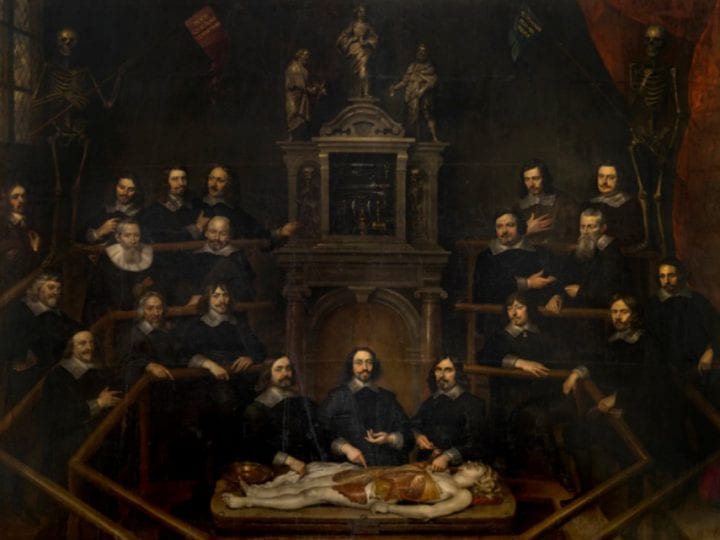The image depicts a very old and detailed painting, likely from the 1700s, presenting a somber and historical scene. Central to the composition is a table with a partially skinned body—displaying a fleshy brownish color from the chest down to the knees, while the rest of the body remains pale and white. Three men, clad in black outfits with white collars, stand directly behind the table, scrutinizing the dissection. Surrounding them is a structured assembly of men, also in black attire featuring wigs, capes, and beards, forming three ascending rows. The first row behind the three central figures consists of five men, the second row houses six men, and the third and final row includes an additional six men. Flanking this macabre scene, a skeleton on both the right and left holds a flag, adding to the grim atmosphere. The backdrop features a large clock or an artistic design, suggesting a possible setting in a medical or governmental institution. The entire painting, done in a dark, old style, captures a moment of scientific or medical examination from centuries past.